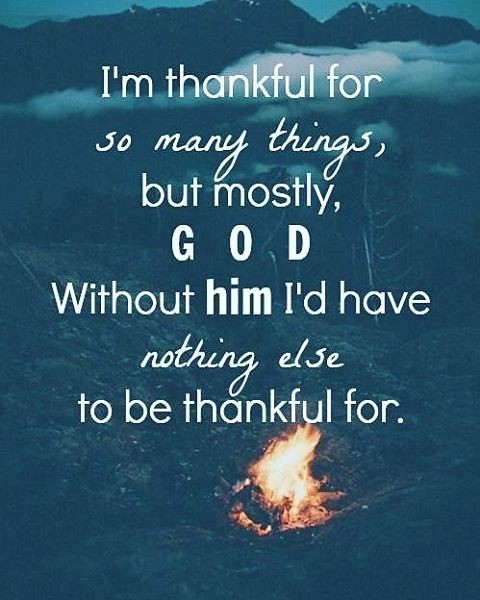The image features an inspirational quote presented in pale blue letters, reading, "I'm thankful for so many things, but mostly God. Without Him, I'd have nothing else to be thankful for." The text is a combination of script for the phrases "so many things" and "nothing else," and regular type for the rest. The background is a faded blue landscape with rolling hills in the foreground, partially visible trees mid-background, and a row of mountains with clouds near the top. A vibrant, bright fire with visible flames is prominent in the foreground, casting the only vivid colors—red, yellow, and hints of white. The overall appearance evokes a sense of reflection and gratitude, suitable as a contemplative poster or piece of wall art.